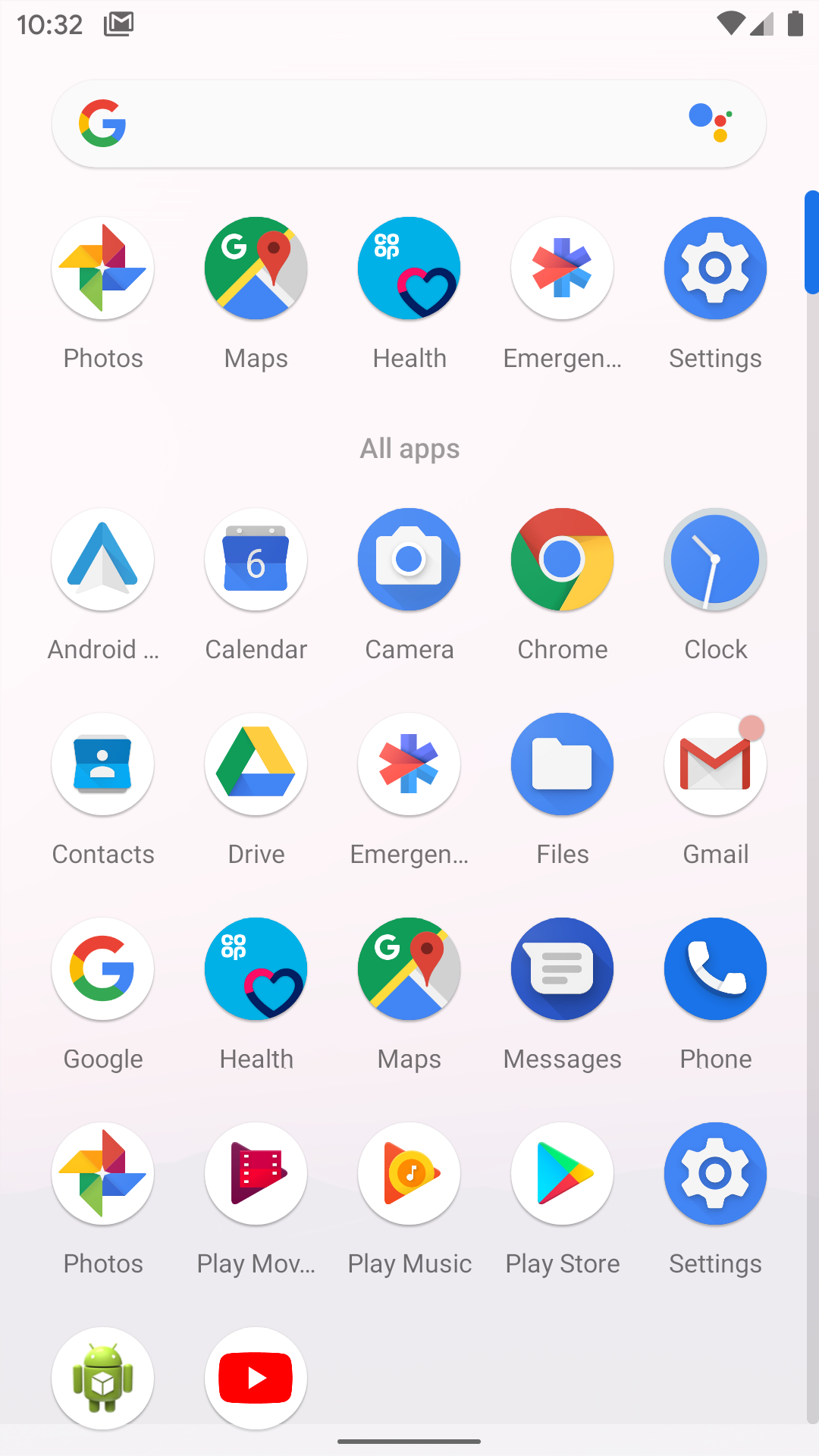This vertical gray image displays a detailed arrangement of various icons and symbols typical of a smartphone interface. The top-left corner shows the time "10:32," along with several status indicators. A mail emblem accompanied by a box is present, followed by a fan icon to the right. Adjacent to these is a partial right-angle triangle indicating the Wi-Fi signal strength. The fully black battery icon signifies a full charge.

Further down the screen, an oblong shape with a bold "G" is visible, indicating a prominent application or feature. A series of dots are aligned below; a blue dot is on the left, directly below which are yellow and red dots stacked vertically, with the red dot being smaller than the yellow. A tiny green dot is placed in the upper right corner among these dots.

On the main interface, five app icons appear in the first row. Starting from the left, the first icon represents "Photos," depicted by a colorful pinwheel. Next, "Maps" is identified by a circular icon with the letter "G" and a map marker. The "Help" app is shown with four white squares forming a larger square that contains a heart, where one lobe of the heart is black. An "Emergency" app follows, featuring a six-pointed star symbol with two shades of blue and a red segment. The final icon, "Settings," is indicated by a blue gear symbol.